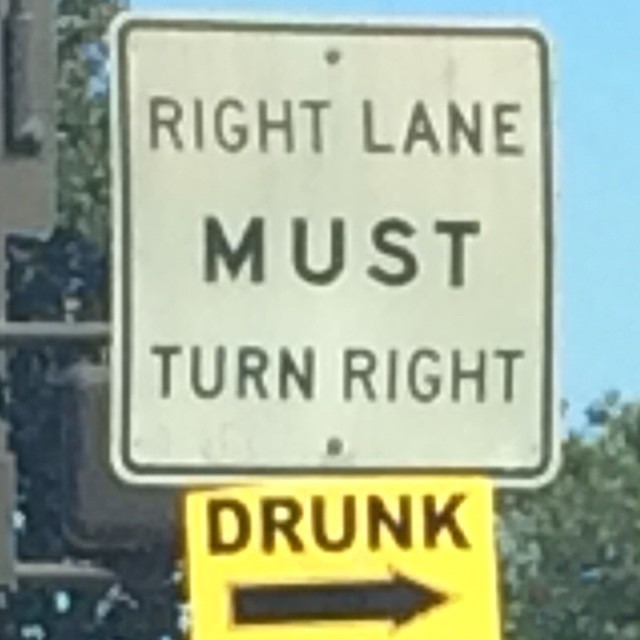This color photograph captures a street sign with a muted palette and slightly soft focus, giving it a vintage or filtered appearance. At the top of the image is a square white sign bordered by a thin black line, which reads "RIGHT LANE MUST TURN RIGHT" in bold black lettering. Directly below, a yellow rectangular sign with black text warning "DRUNK" is mounted, and beneath it, an arrow points to the right. These signs are attached to metallic poles positioned on the left side of the frame. The background features a clear blue sky, and trees are visible both behind the poles on the left and in the lower right-hand corner, extending towards the center of the image.